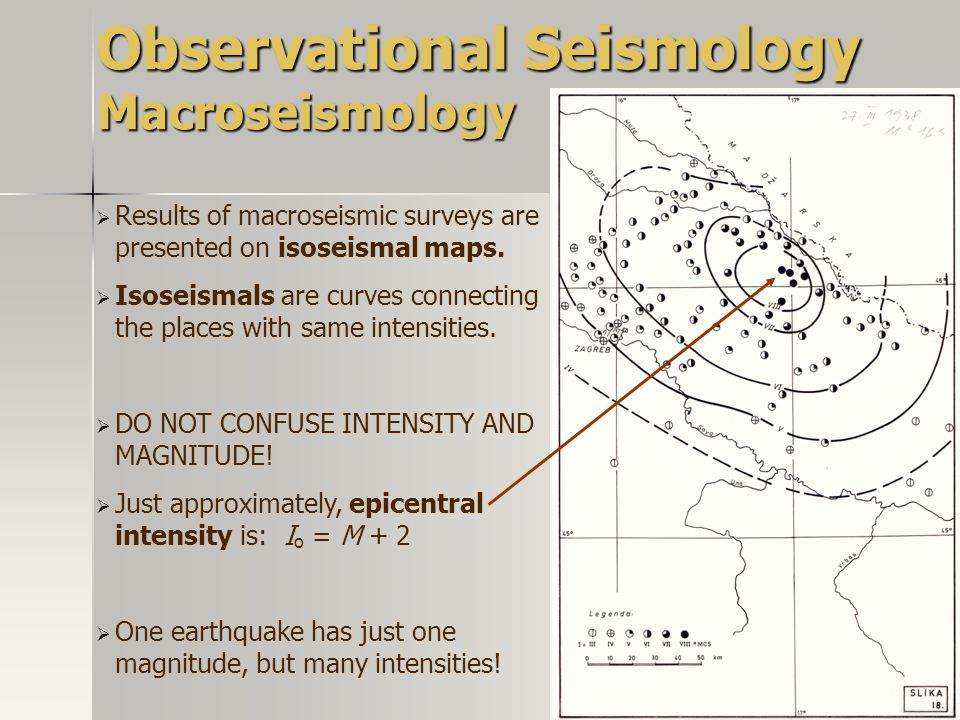This image features a rectangular poster resembling an informational slide from a PowerPoint presentation. The background is gray, and it prominently displays the title "Observational Seismology, Macro Seismology" in yellow letters at the top. Below the title, additional information is presented in dark brown font. 

On the left side of the poster, key points are highlighted, including the presentation of macro seismic survey results and the explanation of isosysmal maps—curves that connect places with the same seismic intensities. The text stresses not to confuse intensity, which can vary across locations, with magnitude, which is a singular value for an earthquake. The poster also features a scientific equation: "Epicentral Intensity (I₀) = Magnitude (M) + 2," and notes that one earthquake can have multiple intensities but only one magnitude.

On the right side of the poster, there is an illustrative map with a white background, containing swirls, dots, and lines to visualize data, including an arrow pointing to one of the dots to indicate seismic activity magnitude. The overall color scheme includes shades of white, black, red, gold, and gray, and the layout design reinforces the educational and scientific theme.